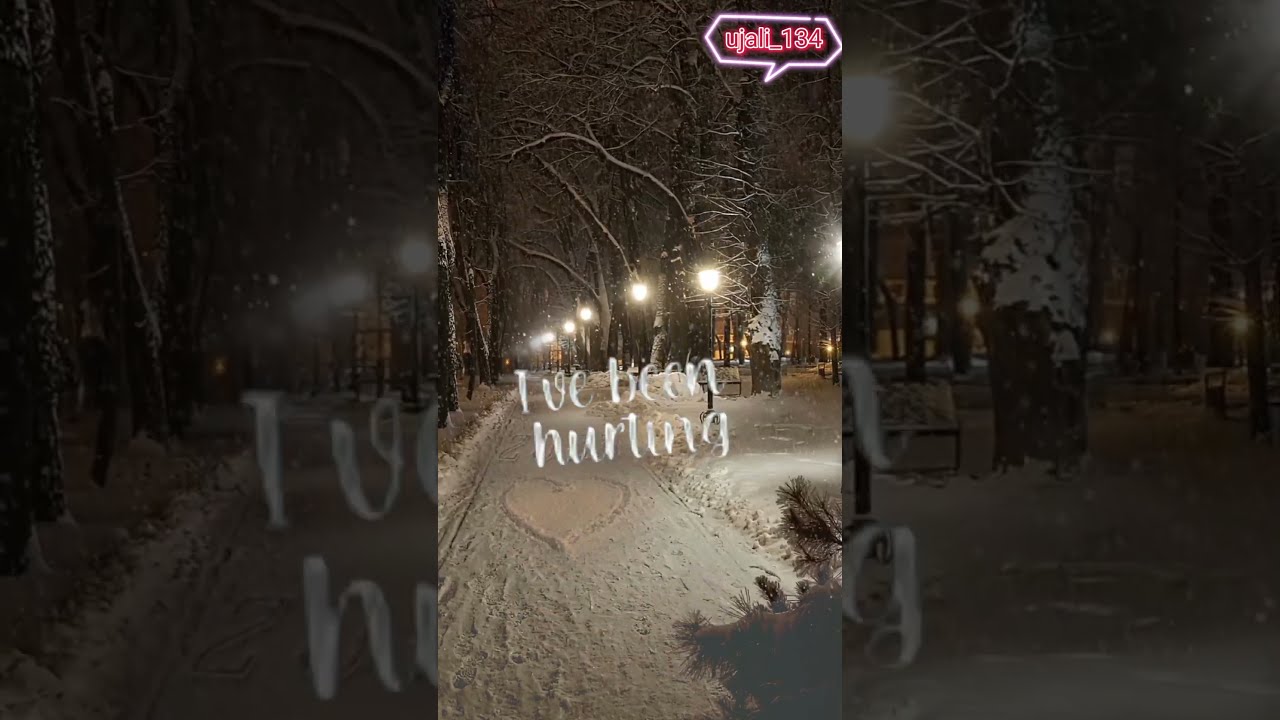This image is a three-paneled, full-color nighttime winter scene. Set within a snowy park, it depicts a central path flanked by dark trees dusted with windblown snow on their trunks and branches. White lights from street lamps on black poles line the path, adding a soft glow to the scene. In the background, hints of additional lights and buildings peek through the trees. At the heart of this serene yet somber scene, a heart shape is etched into the snow of the central path. Overlaying the center of the image in swirling white lettering are the words, "I've been hurting." Additionally, a red speech box in the upper right corner contains peculiar text that reads, "You jail, J-A-I, J-A-L-I - 134."